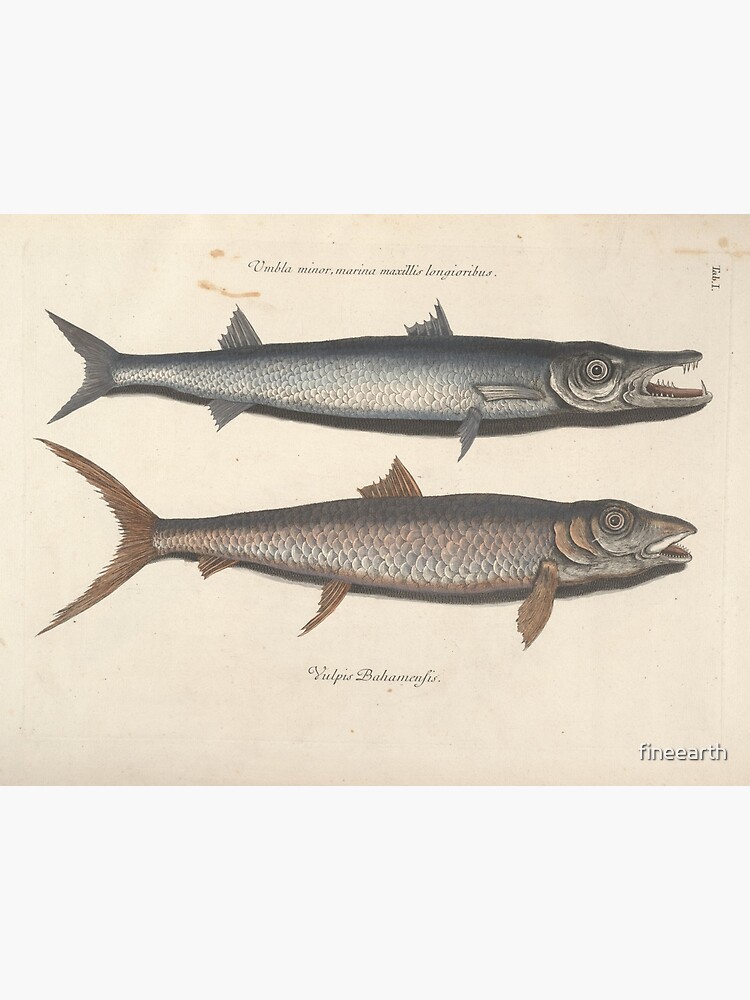The image depicts a piece of vintage wall art featuring two illustrated fish on a slightly discolored, cream-colored background. Both fish are oriented to display their right profiles, laid out horizontally against the white paper. The fish on the top has a longer face and a short tail, is a steel blue-gray color with darker edges and fins, and has sharp, narrow teeth with some gaps. It has its eye wide open. This fish features two fins on top and two on its side, and additional details of gills near its eyes. The fish on the bottom is copper-brown, with a shorter face and longer tail, and boasts solid teeth. It has one fin on top and two on its bottom, along with an eye similarly facing the viewer. There is cursive writing indicating the species of the fish, although the text is too small and illegible to read. In the bottom right-hand corner, the artwork is marked with the words "Vintage Wall Art" in a white font.